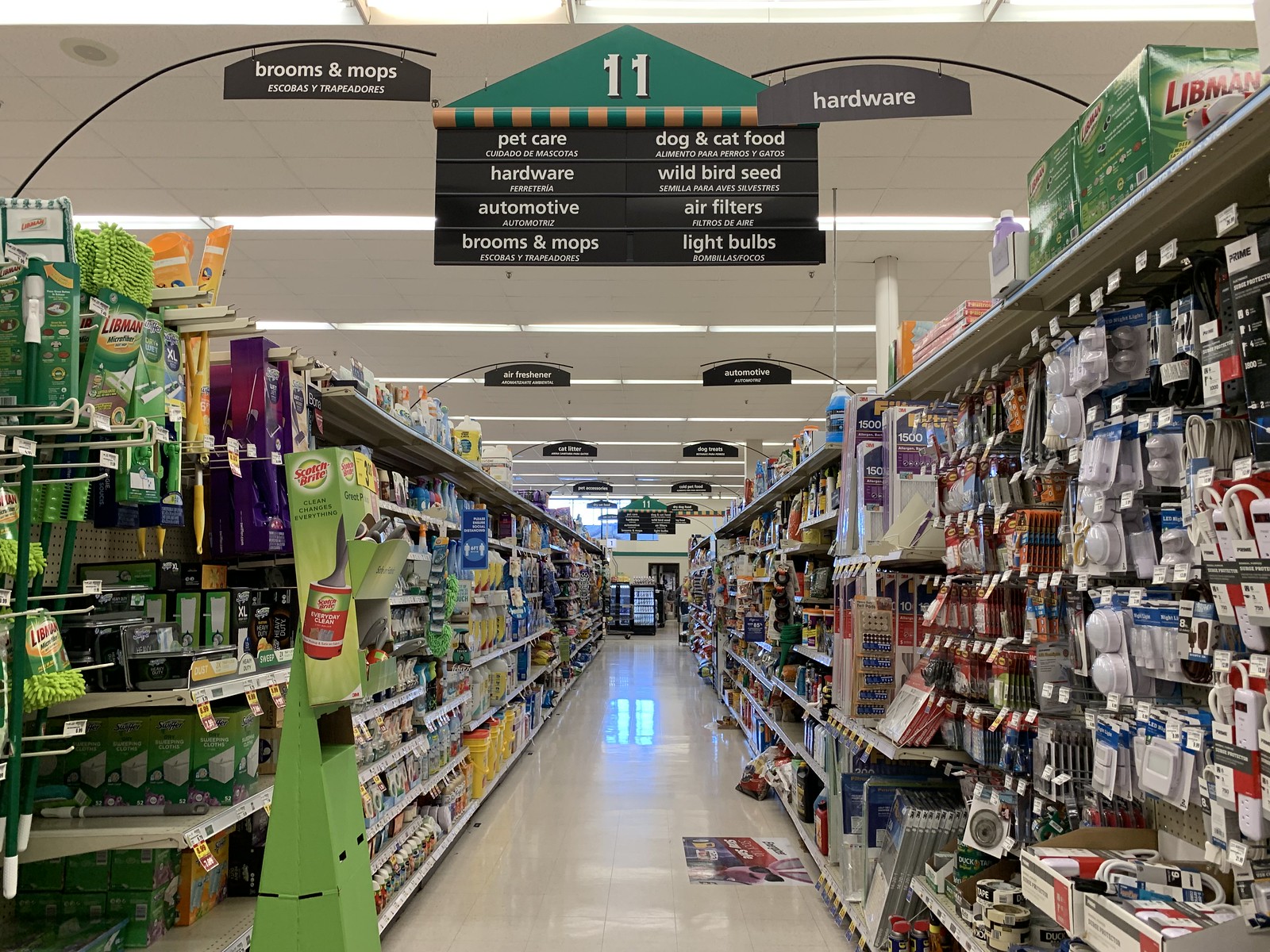The photo, taken inside a hardware store, captures the scene from the end of an aisle looking straight down its length. A prominent sign hangs above the middle of the aisle, labeled "Aisle 11," and lists the categories available in this section: pet care, hardware, automotive, brooms and mops, dog and cat food, wild bird seed, air filters, and light bulbs. On the right side of the aisle, the shelves are stocked with extension cords, various types of lighting, and rolls of tape. The left side displays an assortment of mops and sponges. The aisle floor is plainly visible, extending directly forward, while overhead, a T-bar ceiling with white lighting provides clear illumination.